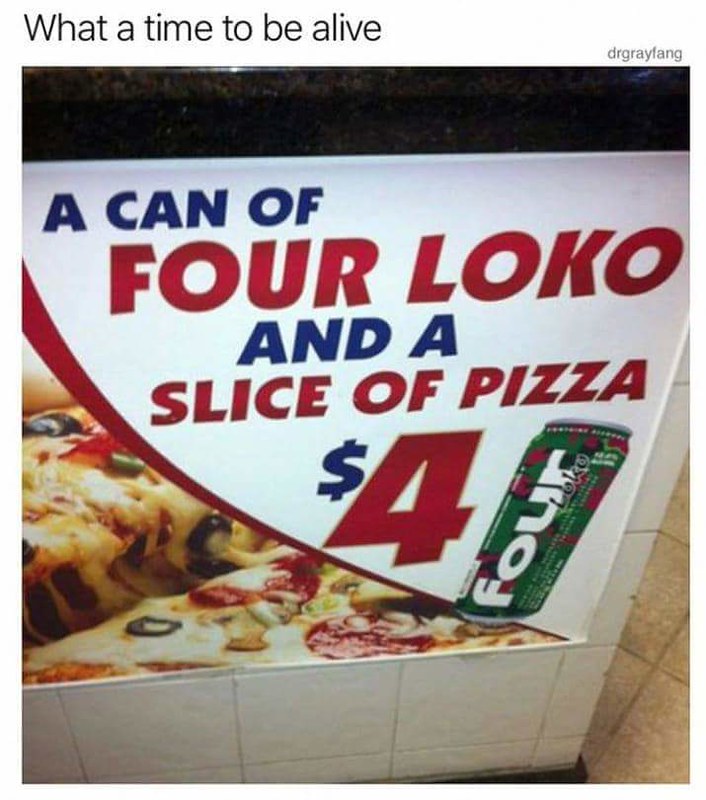This image is a detailed advertisement for a meal deal, seemingly located in a subway environment. The ad prominently displays the tagline "What a Time to be Alive" at the top, alongside the name "Dr. Grave Fang" written as "DrGraveFang" in lowercase letters. The poster features a striking design with a white upper half and a diagonal red, curved line that slices the image from the upper left to the lower right.

The main visual elements are a close-up photograph of a supreme pizza on the left, showcasing a slice being lifted with cheese pulling away, and a green can of Four Loco with white, black, and red accents on the right. The ad's text is boldly displayed in capital letters, stating, "A can of Four Loco and a slice of pizza, $4," with the dollar sign in blue and the number four in red. The overall color scheme of the font alternates between red and blue on a white background.

The setting appears to be on a tiled wall with additional brownish tiles along the floor, suggesting it may be located in a subway station or a similar public transportation area. The image is somewhat blurry but clearly intended to catch the attention of passersby looking for a quick, affordable meal option.